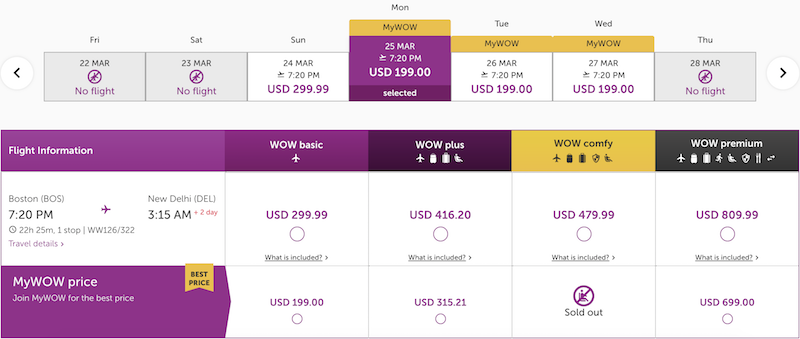**Detailed Caption for Airline Booking Website Screenshot**

The image is a screenshot from an airline booking website displaying various flight options and prices. At the top of the screen, there is a horizontal row listing the days of the week: Friday, Saturday, Sunday, Monday, Tuesday, Wednesday, and Thursday. Each day has an associated date underneath: Friday, 22 March (no flight available); Saturday, 23 March (no flight available); Sunday, 24 March (flight at 7:20 PM, priced at USD 299.99); Monday, 25 March (flight at 7:20 PM, priced at USD 199.99); Tuesday, 26 March (flight at 7:20 PM, priced at USD 199.99); Wednesday, 27 March (flight at 7:20 PM, priced at USD 199.99); and Thursday, 28 March (no flight available).

The date Monday, 25 March, is selected in the screenshot. Below the dates, there is a table with detailed flight information. The selected flight is from Boston to New Delhi, departing at 7:20 PM and arriving at 3:15 AM two days later, with a total flight time of 22 hours and 25 minutes and one stop on flight numbers WW126 and 322. A button labeled "Travel Details" is also visible.

Four different flight options are listed: Wow Basic, Wow Plus, Wow Comfy, and Wow Premium. The prices for these options are USD 299.99, USD 416.20, USD 479.99, and USD 809.99, respectively. 

Beneath the flight options, there is a section displaying the "MyWow" prices, advertised as the best available prices for members. The MyWow prices for the flight options are: Wow Basic at USD 199.99, Wow Plus at USD 315.21, Wow Comfy marked as sold out, and Wow Premium at USD 699.99. There is also an invitation to join MyWow to access these best prices.